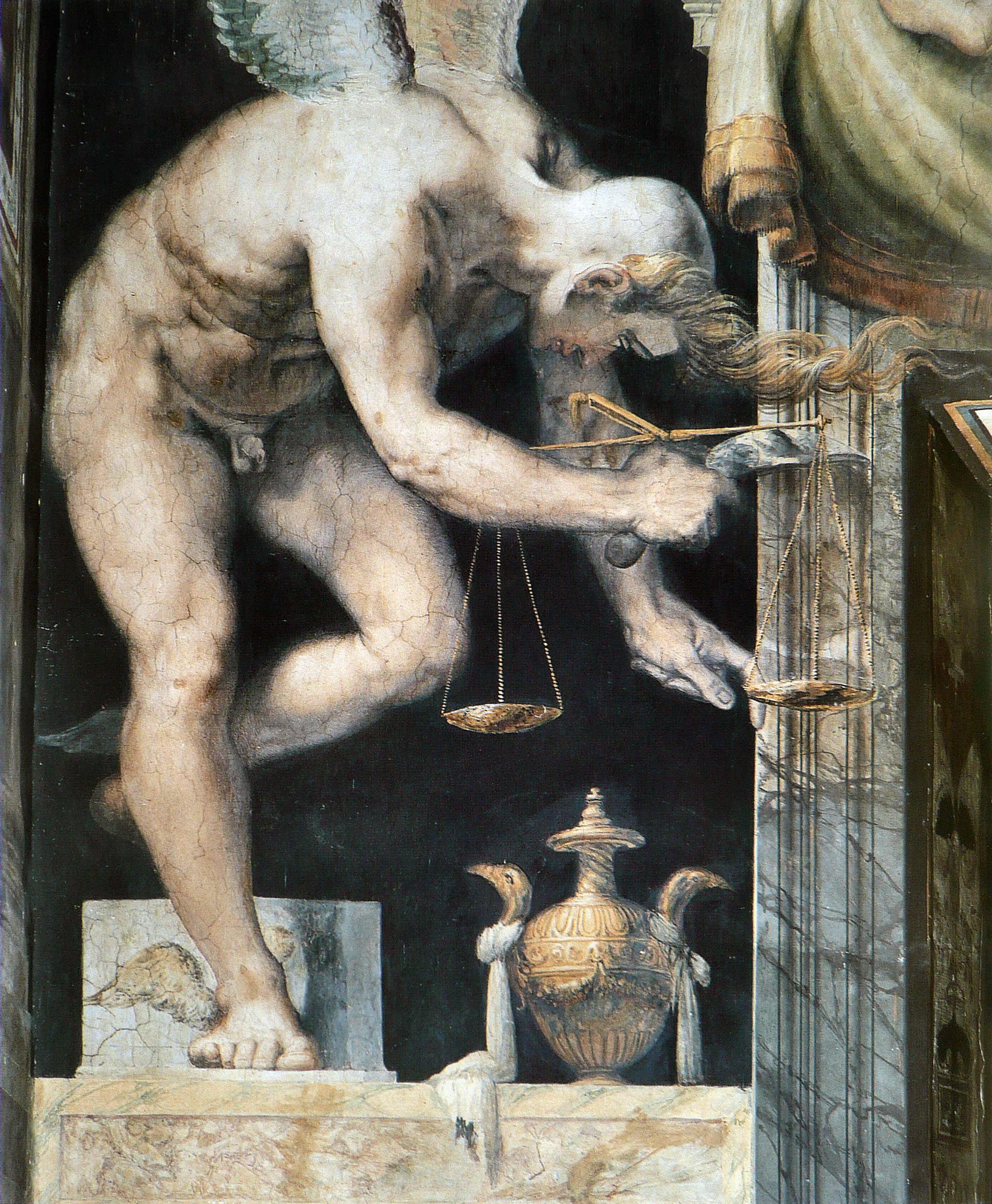The image captures a striking sculpture of a nude male angel, intricately crafted to reveal his muscular physique, complete with visible abs, biceps, triceps, and strong thighs. The angel is bent over, reaching towards the ground with one hand, holding the scales of justice, symbolizing a connection to justice or fairness. His large wings rise majestically from his back, and his hair is long at the front but shaven at the back. He stands supported by one flexed leg on a marble platform with an elaborate golden pot below him, featuring two spouts. To his left, a column draped with green curtains adds a dramatic backdrop, along with a piece of broken cement behind his standing leg. The entire scene is set against a dark background, enhancing the sculpture’s imposing presence and intricate detail.